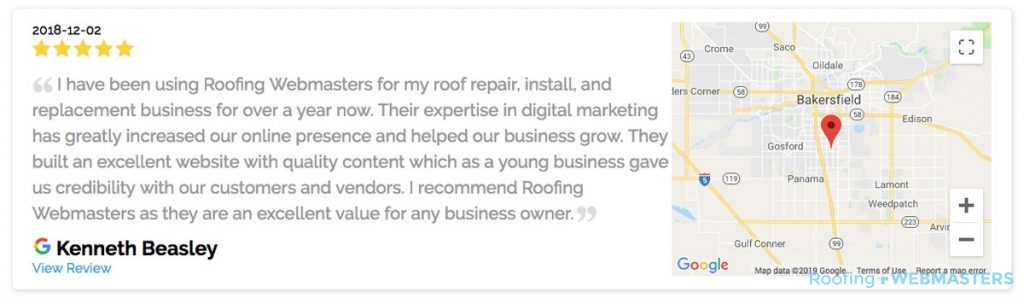Displayed prominently on the right-hand side is a map of Bakersfield, California, featuring a red mark that specifies the location of the company "Roofing Webmasters." The map is presented in a minimized format, providing a general sense of the area rather than detailed specifics. The map interface includes interactive plus and minus icons, allowing users to zoom in and out for a more precise view.

Adjacent to the map on the left is a detailed user review dated December 2, 2018. The review, which received a perfect five-star rating, is attributed to Kenneth Beasley, although his company affiliation is not disclosed. The text of Kenneth's review, enclosed in quotation marks, reads: "I have been using Roofing Webmasters for my roof repair, install, and replacement business for over a year now. Their expertise in digital marketing has greatly increased our online presence and helped our business grow. They built an excellent website with quality content, which as a young business gave us credibility with our customers and vendors. I recommend Roofing Webmasters, as they are an excellent value for any business owner."

Next to Kenneth Beasley's name is the Google emblem, indicating that this review is affiliated with Google Reviews. Additionally, at the bottom of the review, there is an option labeled "View more reviews," though its function—whether to expand the current review or to navigate to additional reviews—is unclear. The map itself is branded with the Google logo in the lower-left corner.